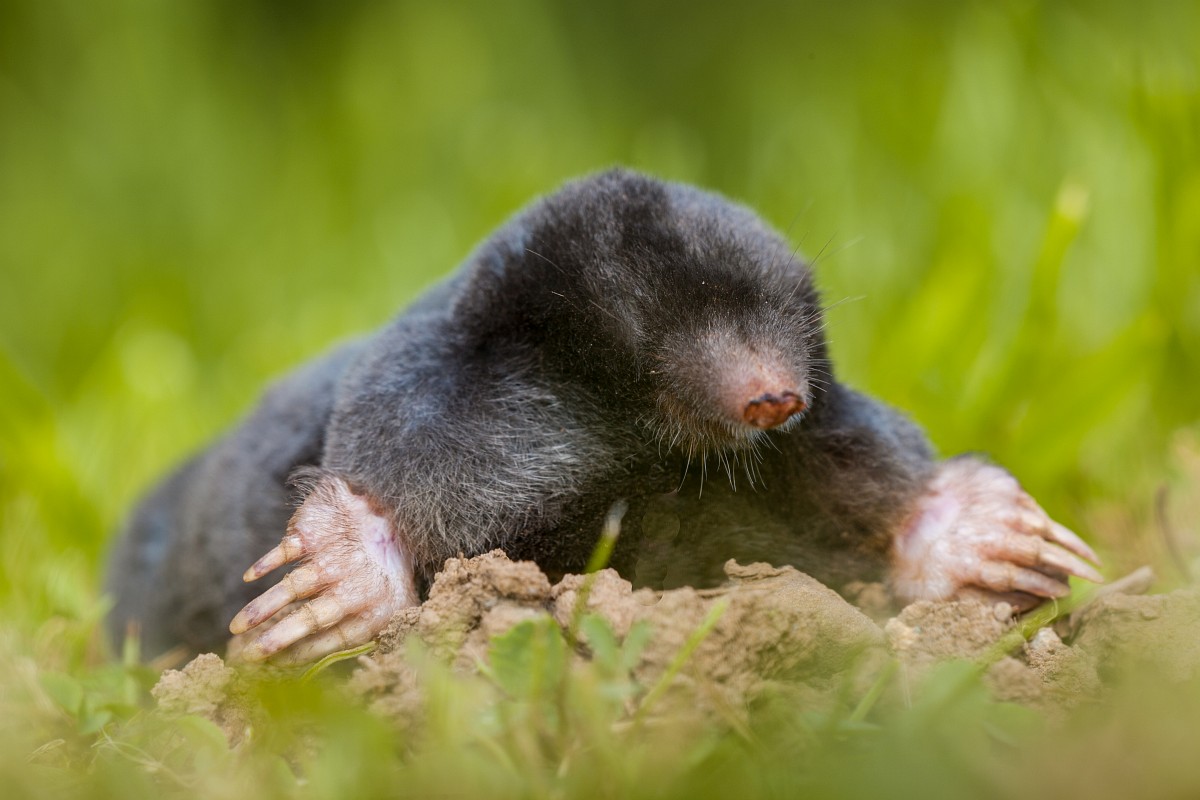The image features a small, incredibly cute mole, characterized by its short black fur and lack of visible eyes, suggesting it might be blind. The mole, covered in dark gray, almost black fur with darker brown-colored nostrils and gray whiskers, is perched atop a lumpy mound of brown dirt, seemingly emerging from a hole or burrow. Its long, flesh-colored hands with off-white, yellowish claws are prominently displayed, indicating its excellent adaptation for digging through soil in search of bugs, insects, and grubs. The background is vividly green with blurry grass both in the foreground and behind the mole, drawing attention to the animal as it surveys its surroundings.